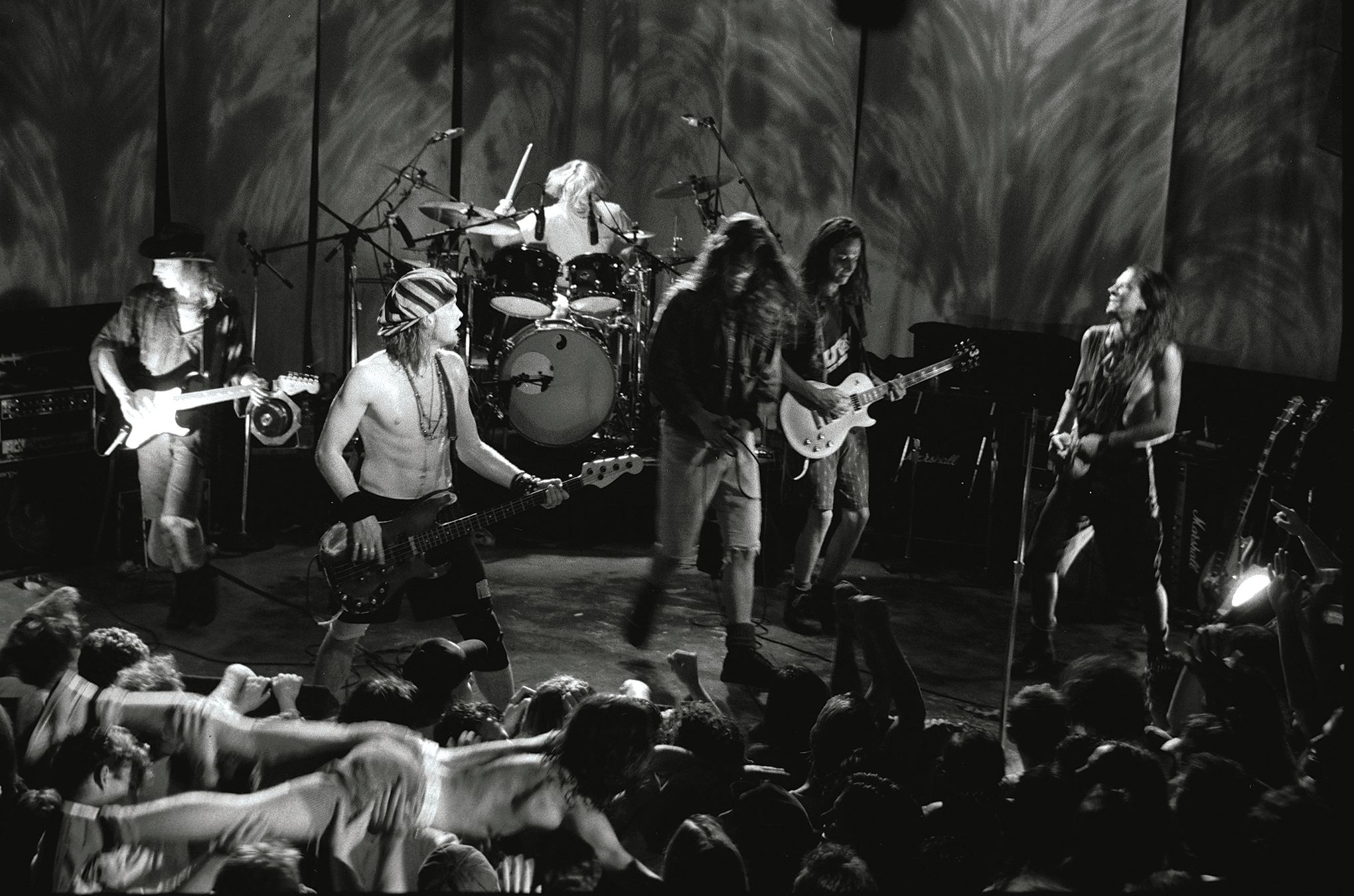In a captivating black-and-white photograph, a rock band of six members electrifies the stage. The rear shows a dynamic drummer, fiercely striking with their right stick raised high as their long blonde hair cascades over their face. Surrounding the drummer are multiple microphones. At the forefront, four guitarists rock out in sync, while a central vocalist—distinguishable by their raised left hand holding a microphone—commands attention without an instrument. The band members are clad in dark, possibly black shirts, blending into the intense atmosphere.

Beneath the stage stretches a sea of enthusiastic fans, tightly packed and exhilarated. Adding to the mayhem, a shirtless and possibly pants-less figure can be seen crowd surfing, their body gliding on outstretched hands from left to right across the lower portion of the image. The background stage décor is shadowy and indistinct, perhaps a folded screen, contributing to the raw energy of the performance scene.